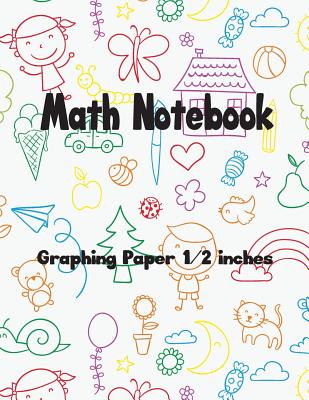The vertically aligned rectangular image is that of a cheerful, child-themed math notebook cover with no border, featuring an off-white background. The top center boasts the bold black title "Math Notebook" in a playful, childlike font. Just below, the text "Graphing Paper 1/2 Inches" is also in black. Surrounding these titles are numerous colorful, outlined doodles of various objects and characters. In the upper left, a smiling girl with her hands out is outlined in red, next to a red butterfly. Nearby, a purple-outlined house and a red heart add to the charm. Further down, a tree in green, a brown-outlined potted daisy, a yellow crescent moon, and a blue cloud are visible. Scattered throughout are additional whimsical drawings, including a girl with pigtails, a boy, a teddy bear, a bumblebee, pieces of candy, fruit, birds, a kitten, a snail, and an ice cream cone. Each illustration is drawn with fine markers in a variety of colors, creating a delightful and inviting design. This cover exudes an inviting, playful vibe, perfect for a child's school supply.